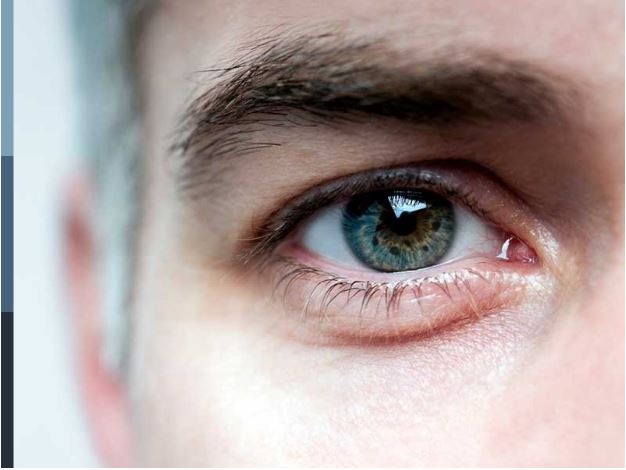This close-up photographic image captures the left eye of an individual with light skin, likely male. The eye is blue with dark blue specks surrounding a black pupil, and there are hints of brown near the pupil. The eye is slightly bloodshot, with a prominent pink tear duct in the inner corner. The eyebrow above is dark and somewhat bushy, while the eyelashes are short; darker at the top and lighter at the bottom. The skin around the eye shows wrinkles and a lighter reflection under the eye, contributing to a pinkish hue. To the left side of the image, parts of the grayish-white hair, including silver and black strands around the ear, are visible but out of focus. The very left edge of the photo features bands of light blue transitioning to medium blue and dark blue from top to bottom. The background across the eye is mainly white and blurred.